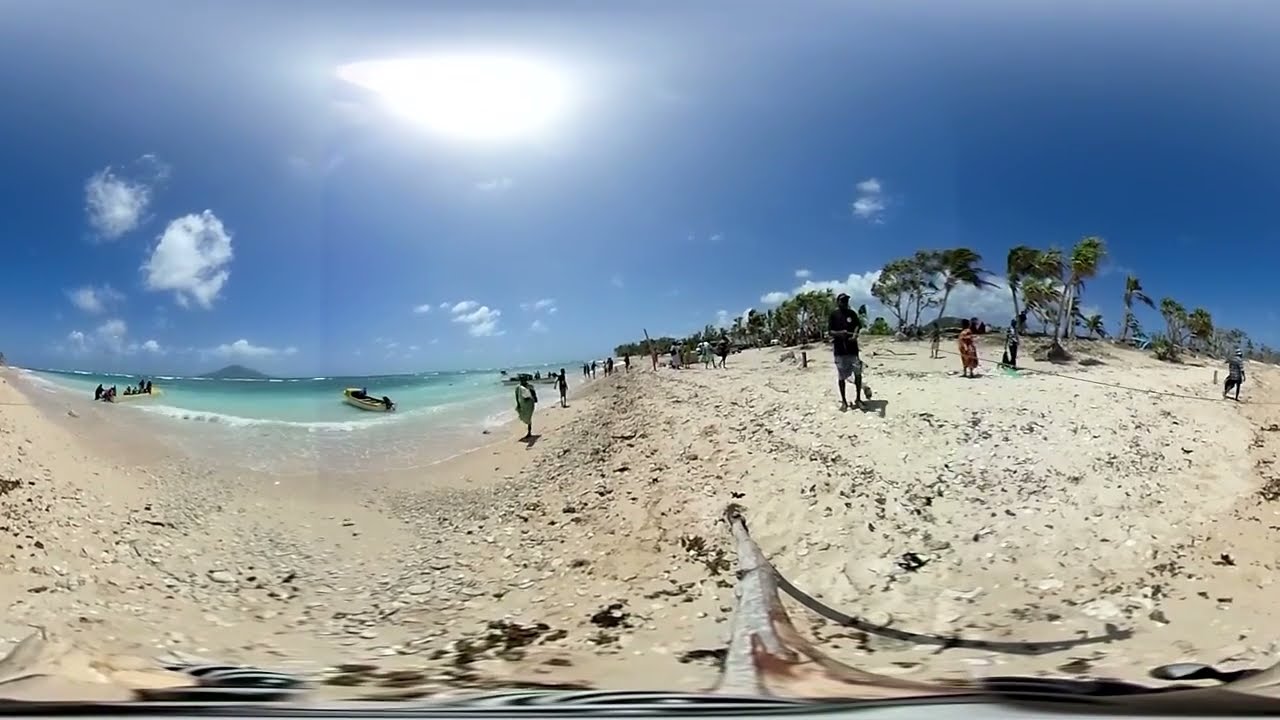Panoramic view of a lively beach scene under a beautiful blue sky with minimal clouds and bright sunshine. The expansive beach has a mix of golden and tan sand, bustling with numerous people walking and jogging. Closer to the water, the sand appears slightly darker in hue. The calm, teal to deep blue water features a small, white rowboat slightly behind the waves. A handful of people are seen on a yellow raft in the water, while another group is positioned on a small sandbar, surrounded by a dozen or more beachgoers. The shoreline is bordered by a dense row of green leaf trees, creating a vibrant backdrop. Scattered along the beach are indistinct items, adding to the typical, energetic beach day atmosphere.